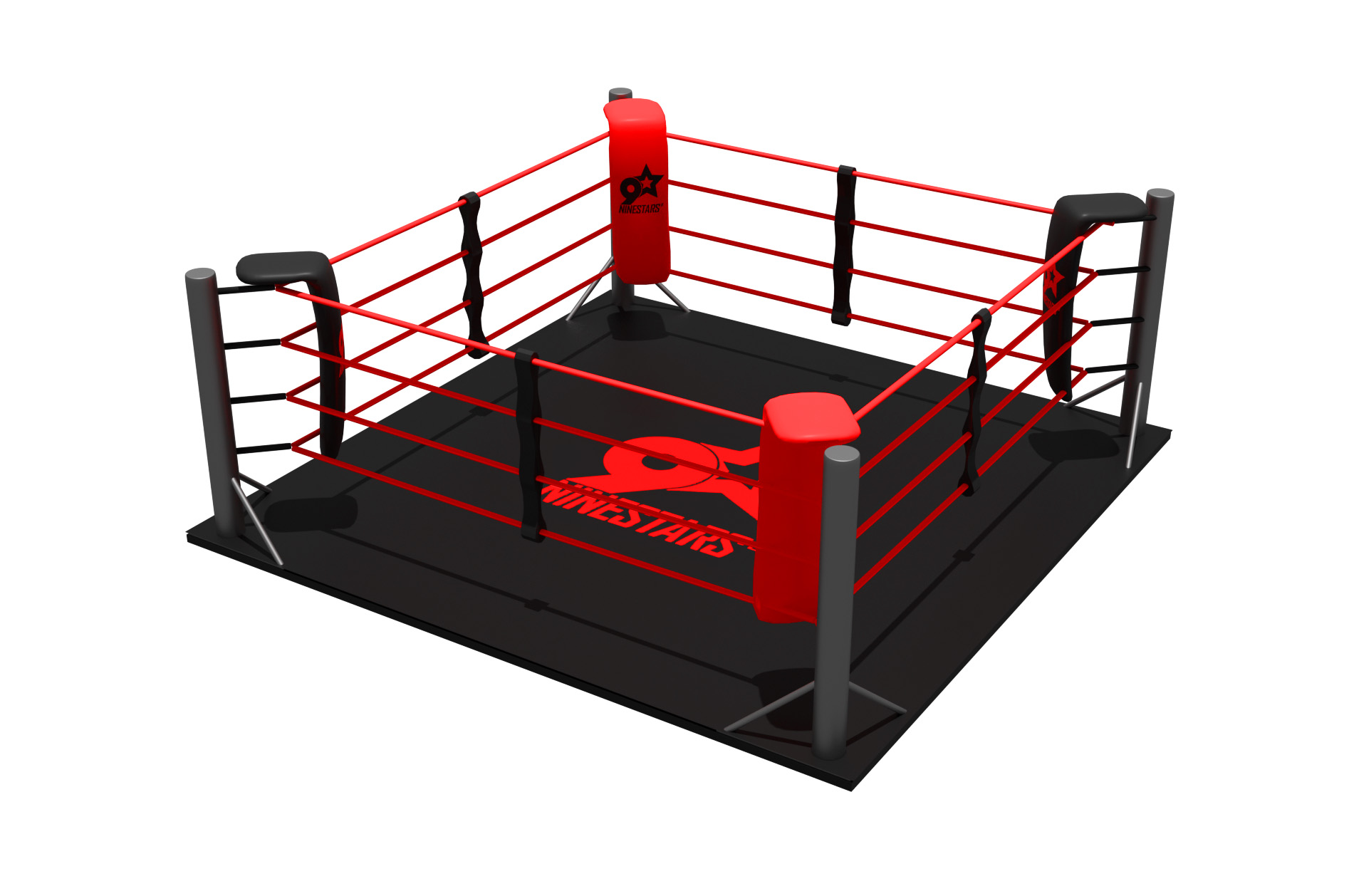The image depicts a computer-generated graphic of an indoor boxing or wrestling ring, likely a product image. The ring is square-shaped and appears to be set against a plain white background, emphasizing the ring itself. Each corner of the ring features a gray post topped with a cushion—two are red and two are black. The red cushions and some black ones prominently display a logo featuring a numeral nine with an attached five-point star, and the text "Nine Stars" below. Surrounding the ring’s perimeter are red ropes connected by shorter black ropes to the posts. The mat inside the ring is black, and in its center is a large version of the same "Nine Stars" emblem, with the numeral nine and a five-point star. The perspective of the image is as if viewed from above and behind the ring, providing a clear view of the arrangement and design details, including the red and black color scheme and branding elements. The scale suggests that this ring could be a toy or a miniature model, as it doesn't appear to be particularly large.